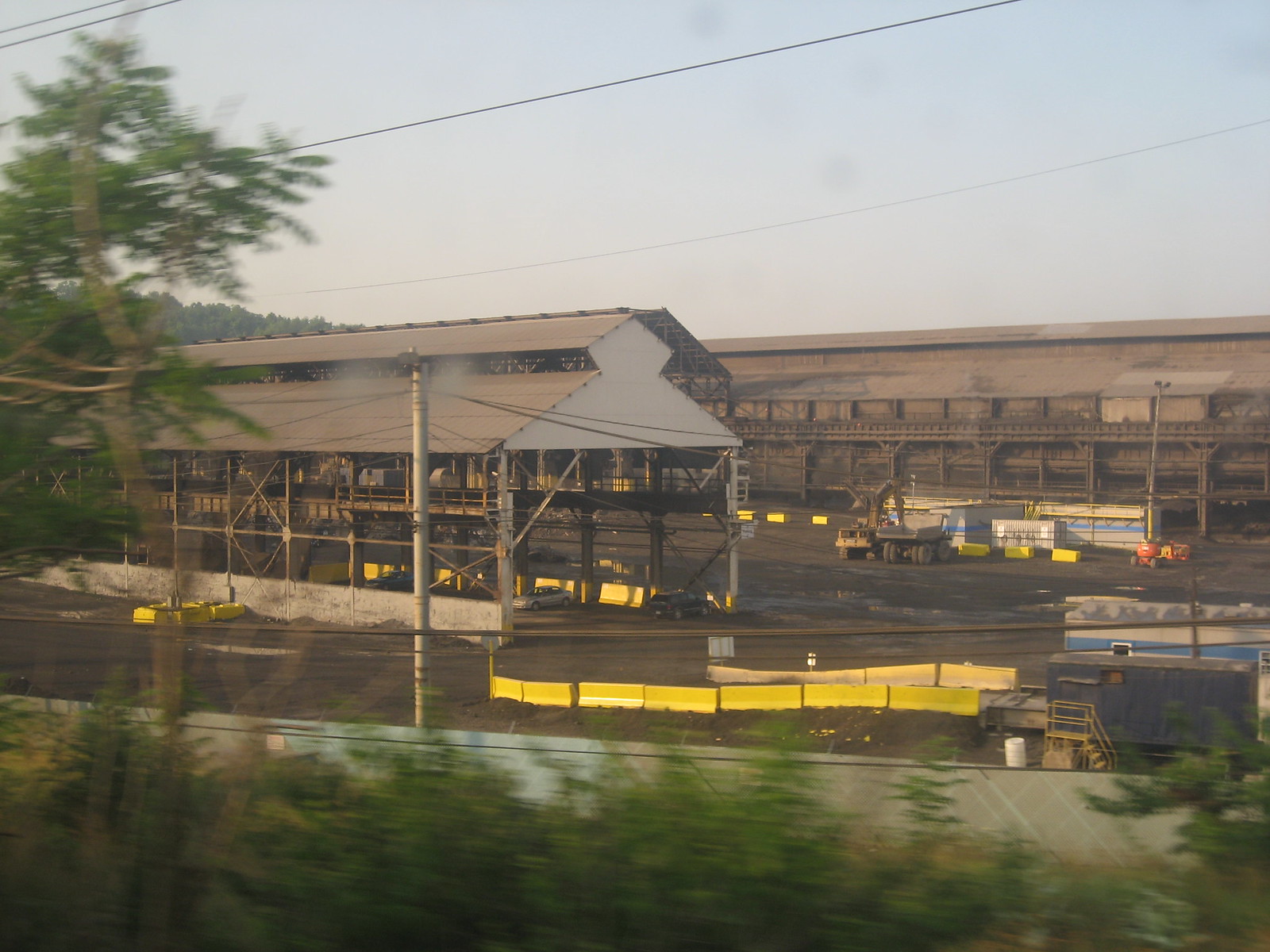This photograph captures a large, weathered industrial area, possibly a construction yard or dock, seen from a moving vehicle, as evidenced by the slight blur around the edges. The area features several buildings constructed from tin and metal, displaying signs of wear and tear. Prominently placed throughout the scene are numerous yellow barricades and dividers that guide vehicles, including a few parked cars underneath a tin-roofed structure and large construction trucks and equipment in the background. The dirt and mud ground further emphasize the rugged, utilitarian nature of the setting. Towards the bottom left of the image, large green trees are visible, adding a touch of nature to the otherwise industrial landscape.